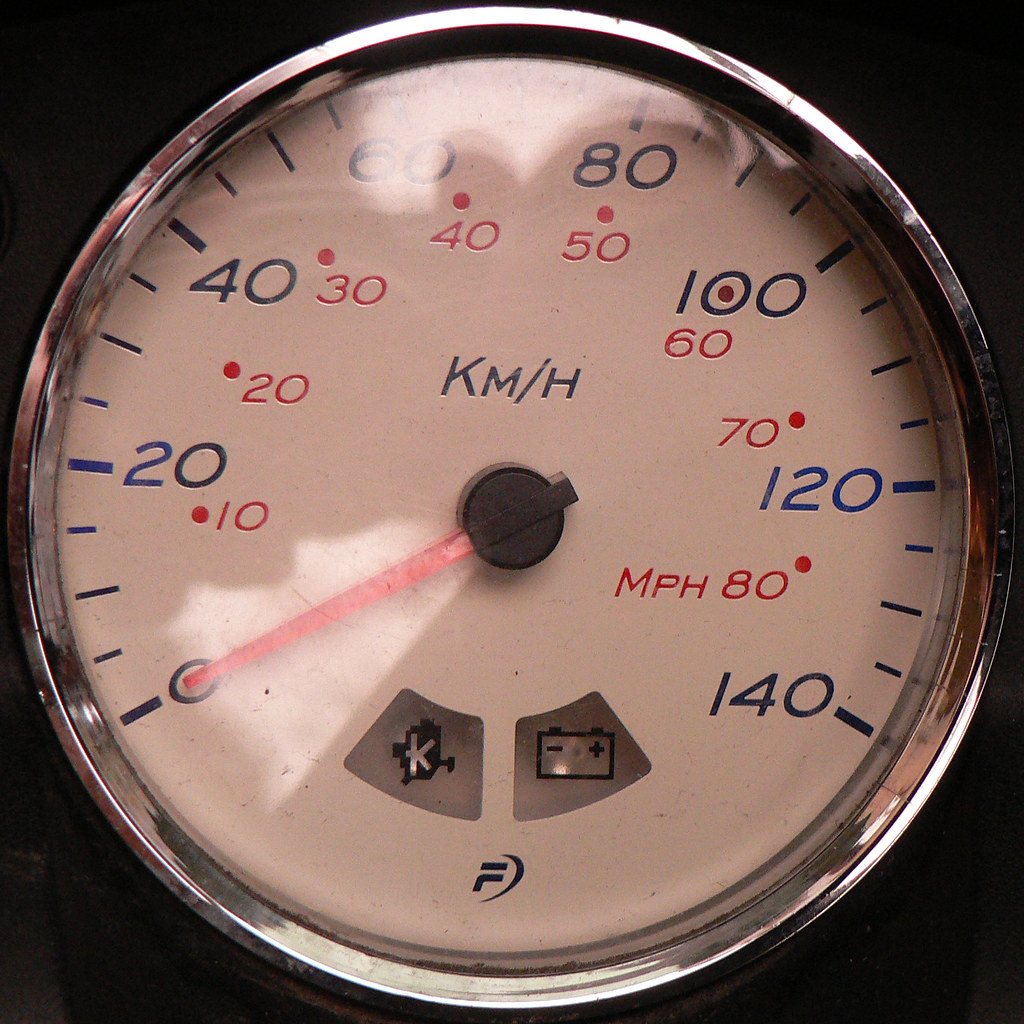This image portrays a detailed view of a gauge. The primary feature is a red needle, prominently resting at the zero mark, indicating no current measurement. The gauge's scale begins at zero and is marked by increments of twenty, with major divisions at 20, 40, 60, 80, 100, 120, and 140, all displayed in dark blue. Between these major divisions, smaller red dotted numbers denote intervals of ten (10, 30, 50, 70, 90, 110, 130), each accompanied by a small dot.

At the bottom of the gauge, there are two small windows. The left window displays the letter "K," while the right window features a box with two knobs labeled "-" (minus) and "+" (plus). Centrally positioned above the needle's pivot point are the letters "KM/H," indicating that the gauge measures in kilometers per hour. A distinctive logo, resembling an "F" combined with a backwards "C," is also visible in blue.

The gauge's background is a clean white, contrasted by a shiny silver chrome outer rim that adds a touch of elegance. The area surrounding the gauge is black and creates a stark contrast, enhancing the readability and focus on the gauge itself.